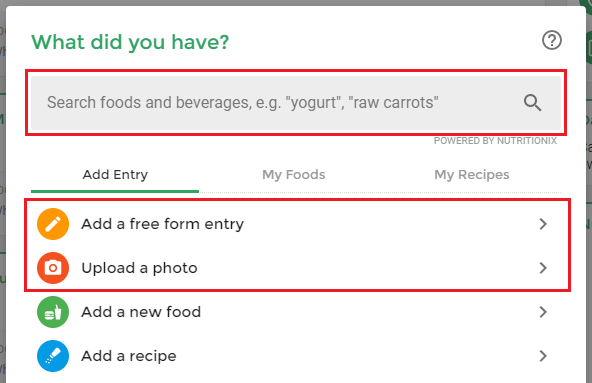The image appears to be a screenshot from a food-related app or website, showcasing a pop-up panel overlaying the main interface. While the background is partially visible, it is largely obscured by the panel. The panel itself is predominantly white, featuring green text at the top that reads, "What did you have?" accompanied by a gray question mark inside a circle.

Below that heading is a gray search field with a magnifying glass icon. The placeholder text in the search field instructs users to "Search foods and beverages, e.g. yogurt, raw carrots," and is outlined in red.

The panel also includes menu options such as "Add Entry," "My Foods," and "My Recipes." "Add Entry" is emphasized, being both bolded and underlined in green.

Under "Add Entry," there are several options outlined in various colors:
1. **Add a Free Form Entry**: Indicated by an orange circle containing a pencil illustration.
2. **Upload a New Photo**: Marked by a red circle featuring a camera icon.
3. **Add a New Food**: Denoted by a green circle with icons of a burger and a drink.
4. **Add a Recipe**: Represented by a blue circle with an icon resembling either a salt or pepper shaker.

Each option has a right-pointing arrowhead at the end. Notably, the "Add a Free Form Entry" and "Upload a New Photo" options are grouped together, enclosed by a red outline matching the search bar.